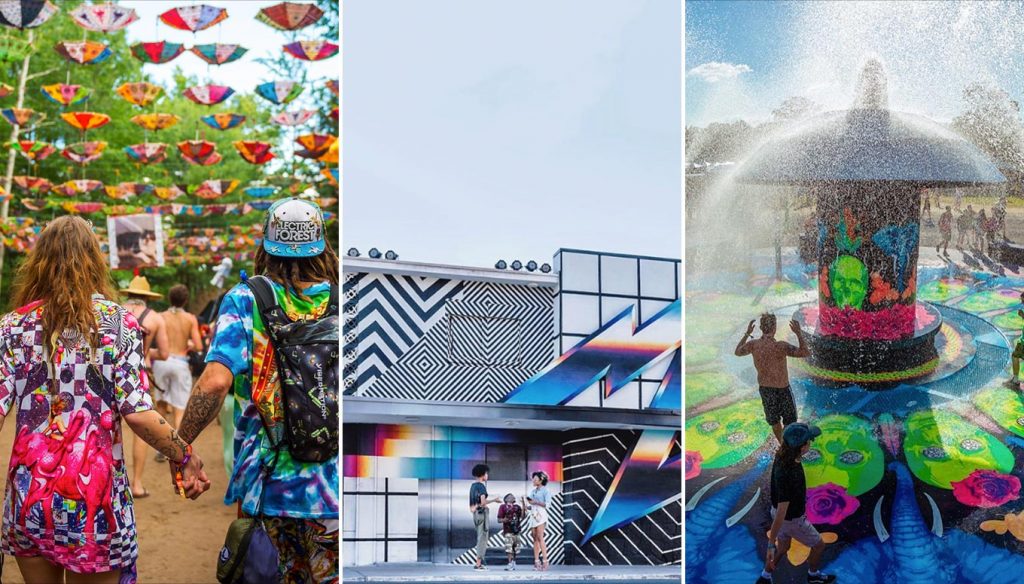The image is a vibrant, three-in-one collage showcasing a lively event at a colorful park. On the left, two individuals—one wearing a tie-dye shirt in blue, orange, and green, with patterned pants and a black backpack adorned with black and white designs, and a hat with blue and white sections; the other in a pink and black checkered shirt with splashes of purple—hold hands under a canopy of upside-down umbrellas strung across the sky in bright hues of blue, red, green, and white. This segment of the picture is bursting with vivid colors like pink, purple, black, white, and orange. The middle section displays a monochromatic, patterned building facade featuring zigzag lines and black and white squares under clear blue skies. Lastly, the right-most image depicts an amusement park scene with a playful atmosphere, where water is spraying from a fountain-like structure surrounded by shades of green, blue, purple, orange, and pink, perfectly capturing the energetic and psychedelic vibes of the park.